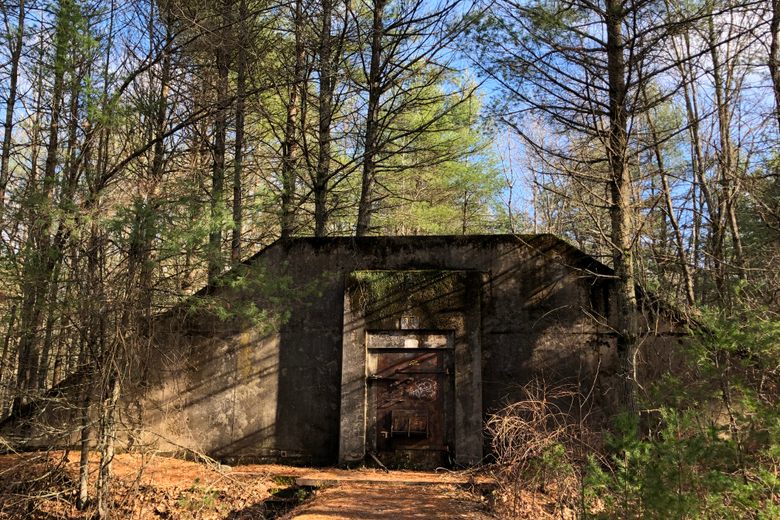In the midst of a dense pine forest, there stands an old, weathered bunker with a strikingly reinforced concrete entrance. The structure resembles a hefty cube with a flattened pyramid top, blending seamlessly into the environment with its moss-covered exterior. At the center of the photo, the bunker’s rusted brown metal door, framed by thick concrete, stands closed, its massive steel hinges still intact. The surrounding forest is lush with very tall pine trees, punctuated by a few dead, gray-barked trees and green bushes that pepper the foreground. Above, the crystal-clear blue sky peeks through the thick tree canopy, hinting at the timeless solitude of this hidden relic. A dirt path meanders towards the door, emphasizing its longstanding presence amidst nature's reclaiming embrace.